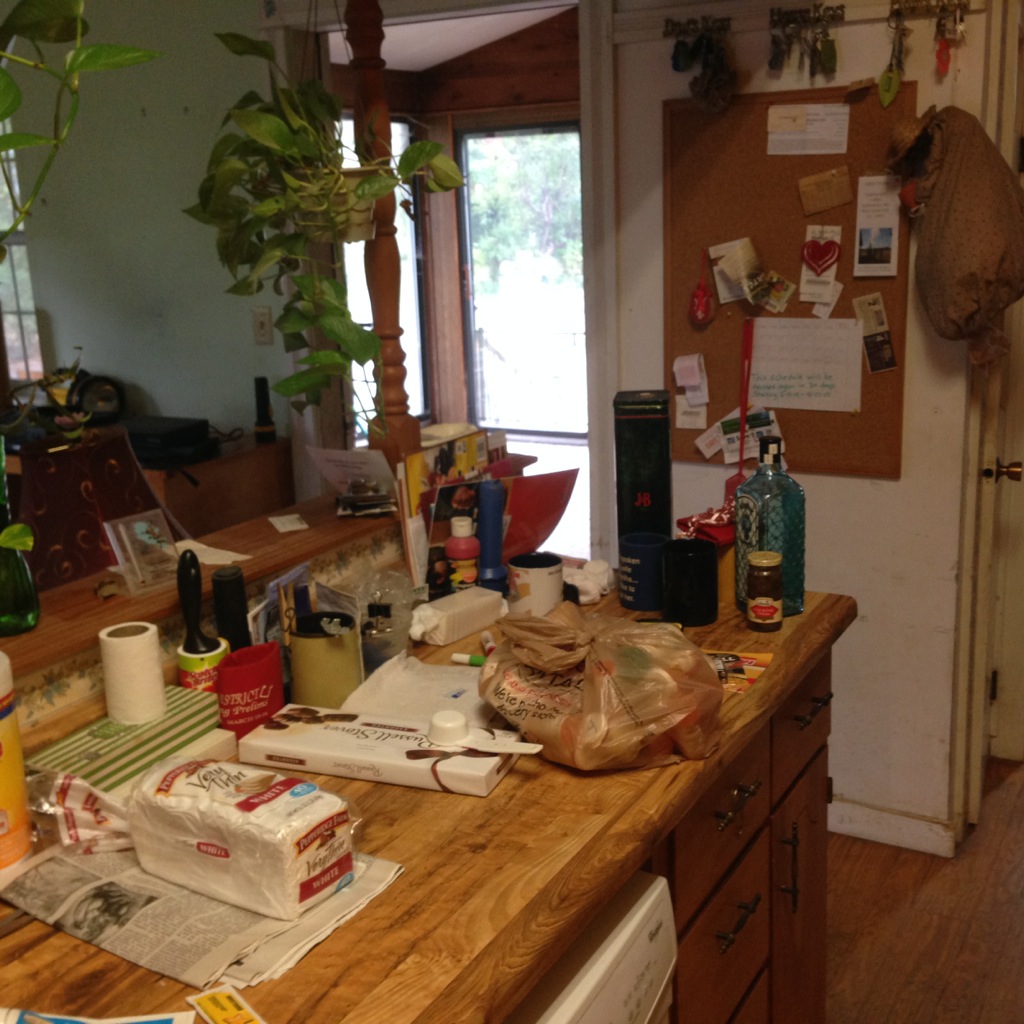The image depicts a well-furnished meeting or demonstration room within a residence, featuring a blend of contemporary and rustic elements. The space is anchored by medium brown wood plank flooring and complemented by pristine white walls. Near the doorway, which is located midway up the right side of the image, a vertical cork board is mounted on the wall, offering a practical spot for notes or reminders.

Adjacent to the entrance stand elegantly crafted turnpost columns, finished in either white or brown wood. Hanging from above is a basket brimming with lush, large-leafed greenery, adding a touch of nature to the interior. 

Dominating the center of the room is a beautifully crafted wooden desk. Atop the desk lies a loaf of bread resting on a newspaper, accompanied by a box of Russell Stover chocolates. Nearby, a brown plastic bag, securely tied, hints at concealed contents. Also present on the desk is a large green cylindrical bottle with a gold cap, a jar of what appears to be jelly or jam, and a package of saltine crackers tucked into the corner. A file holder, filled with articles and file folders, adds to the desk’s functionality.

To the left and further into the room, additional countertops or tables are visible, adorned with planters, an acrylic square frame, white papers, and what seem to be computers or screens, suggesting a versatile space geared towards both work and display.